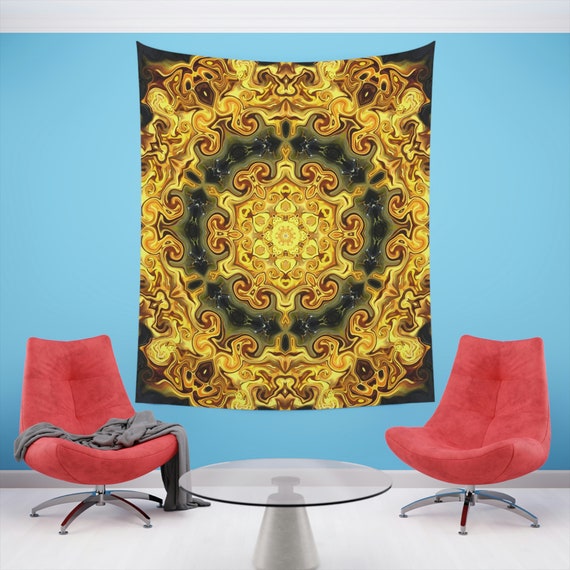The photograph captures a cozy, inviting room characterized by a vibrant blue wall adorned with a large, gold and black tapestry featuring an intricate design that evokes a Versace-like style, though it is not Versace. The tapestry, which is significantly large and nearly covers three-quarters of the wall, is perfectly centered between two plush, burnt cherry-colored chairs. These chairs, which are high-backed and cushioned without armrests, rest on a silver base with tiny rolling wheels. Draped casually over the left chair is a gray blanket that cascades down to the floor, adding a touch of casual comfort. Situated between the two chairs and slightly in front of them is a short, round glass table on a gray platform. The room's flooring is a mix of gray and white, and the atmosphere suggests a space ideal for intimate conversations, podcasting, or interviewing.